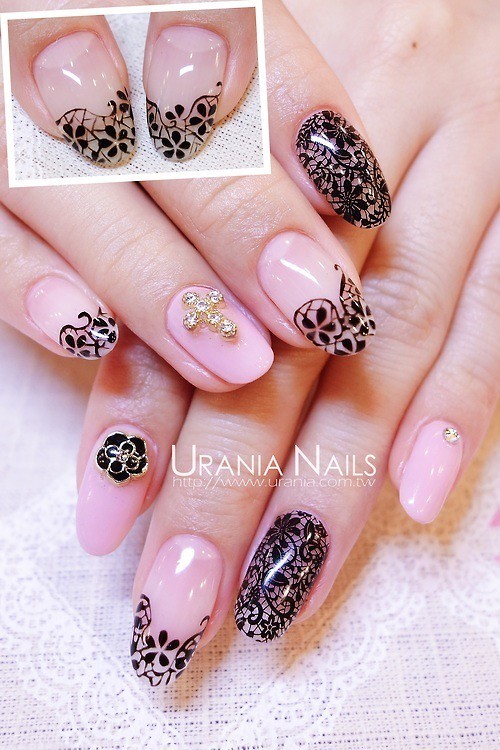This tall, rectangular advertisement for Urania Nails showcases a stunning array of intricately designed fingernails. The primary image features two overlapping hands laid elegantly on a lace surface, positioned diagonally from the top corners towards the bottom. The nails, painted in a delicate pink hue, exhibit a variety of designs in black and gold. Among these, you'll find a striking gold cross, a black lace-like pattern, and a subtle diamond dot. There is also an inset photograph in the top left corner displaying close-ups of the thumbs, which are adorned with black four-leaf clovers on their pink tips. The ad is accentuated by the bold white text "Urania Nails" and their website link, http://www.urania.com.tw, prominently displayed in the center. This enticing visual captures the essence of exquisite nail artistry.